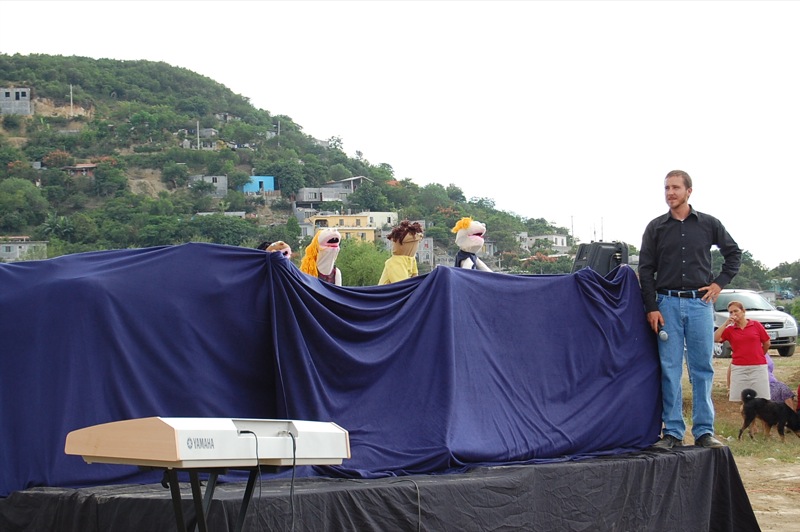The photograph captures an outdoor puppet show on an overcast day. In the foreground, a white Yamaha keyboard rests on a black stand in the lower left-hand corner. Dominating the lower section of the image is a black stage draped in cloth, with a blue vertical curtain serving as the backdrop for the performance. Peering over the curtain are four hand puppets: two boys, one girl, and a pet. The puppets are distinctively designed with two white puppets, one black puppet, and a pet.

Standing on the right edge of the stage is a man with short brown hair and a light complexion. He is dressed in blue jeans, a black long-sleeved button-up shirt, a black belt, and black boots. He has a short mustache and is holding a microphone with a black base and light gray top in his left hand. His gaze is directed to the left. Behind him stands a woman with short brown hair, wearing a short-sleeved red shirt and a white skirt, accompanied by a black dog with chocolate brown legs.

In the background, the scene is set against a large hill adorned with green vegetation and various houses, under a bright but gray sky. A white car is also visible in the background. The ambiance suggests a rural setting with an audience enjoying the charming puppet show.